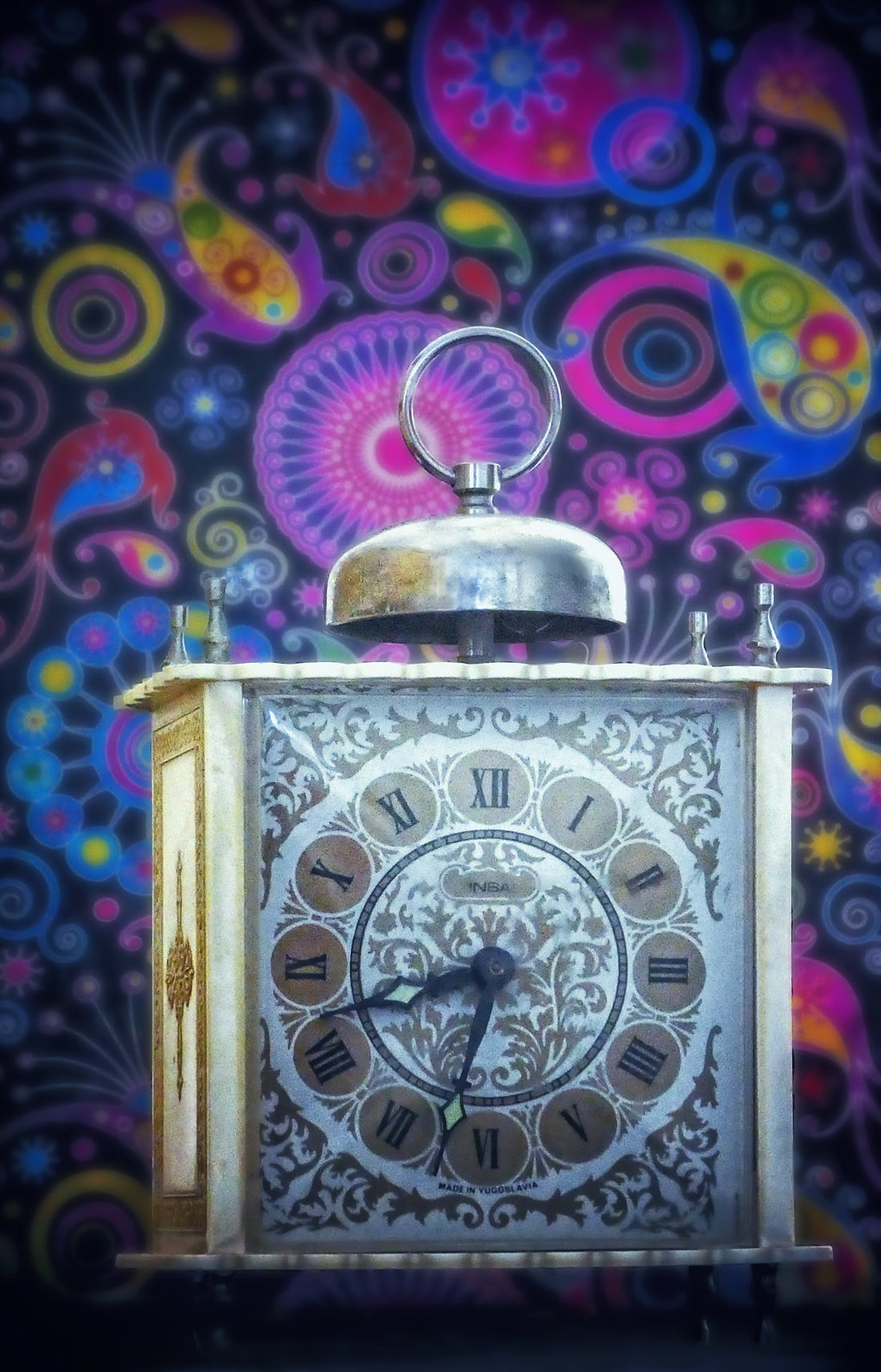An antique alarm clock crafted from faded brass, complete with a prominent bell perched atop it. The clock's design includes a ring, allowing it to be hung on a wall. Its face is adorned with Roman numerals, indicating the time at 8:23, and features an opulent gold leaf background. The clock is encased in a large, ornate casing that contrasts with the modern, eye-catching wallpaper behind it. The wallpaper showcases psychedelic symbols, circles, and swirls in a dazzling array of bright and vibrant purples, pinks, yellows, and blues, creating a striking juxtaposition between the vintage timepiece and its contemporary setting.